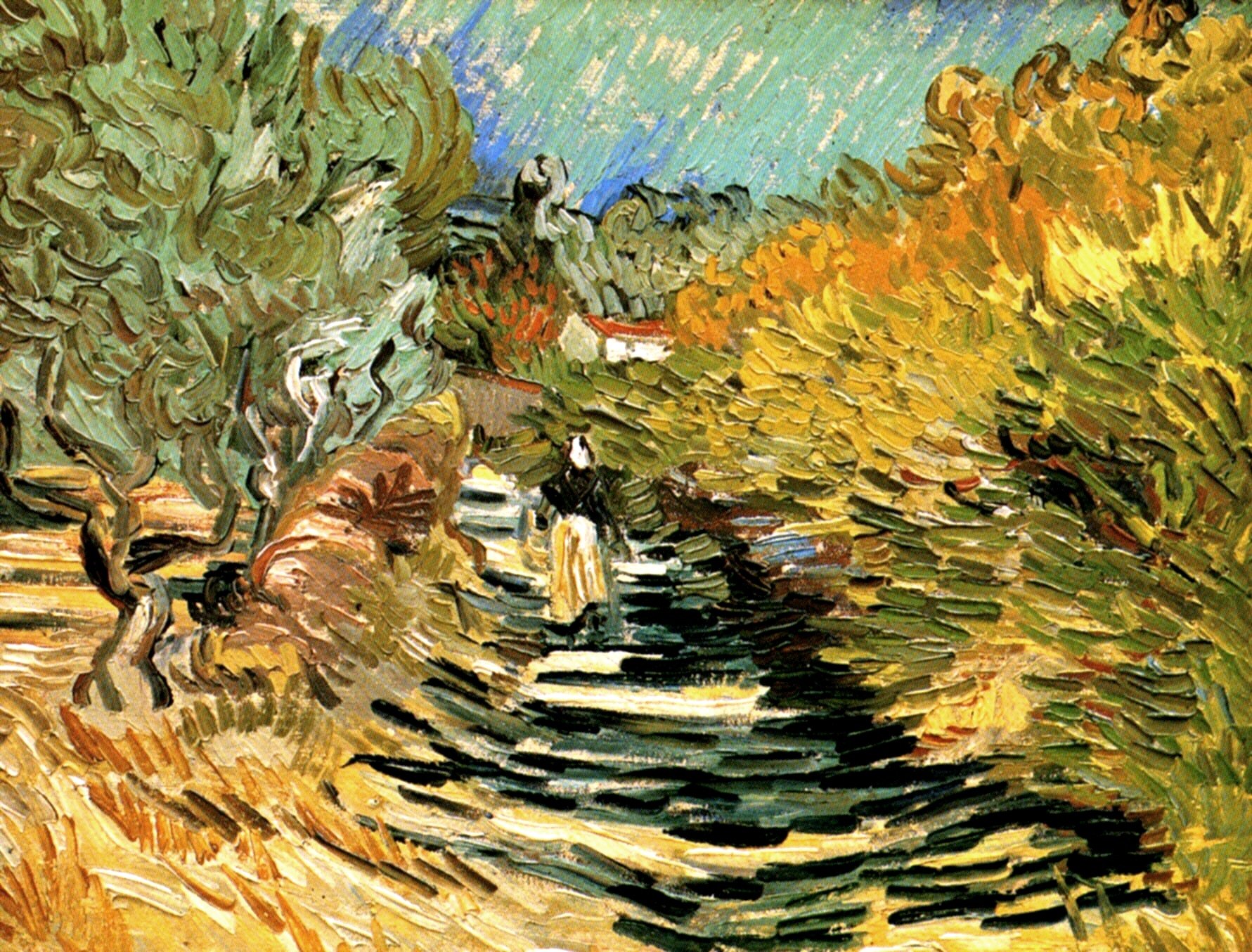The painting depicts a woman walking towards the viewer down a path that features a blend of green, black, and yellow colors. She is attired in a black long-sleeved top and either a blue or gold skirt, her face shown as a white oval with no features. The path is flanked by greenery: on the left side, there are green trees with some yellow underbrush, while the right side showcases a variety of plants in shades of green, yellow, and orange. In the background stands a white house with a distinct red triangular roof, set against an abstract sky composed of green and blue hues with hints of white, blue, and teal streaks. Additional artistic elements include an impressionistic depiction of distant mountains in shades of gray. The brushstrokes are thick and pronounced, giving the painting a slightly three-dimensional and textured feel, embracing its identity as a creative interpretation rather than striving for hyper-realism. The palette encompasses a wide array of colors, including black, white, gray, silver, brown, red, orange, blue, olive, yellow, and tan.